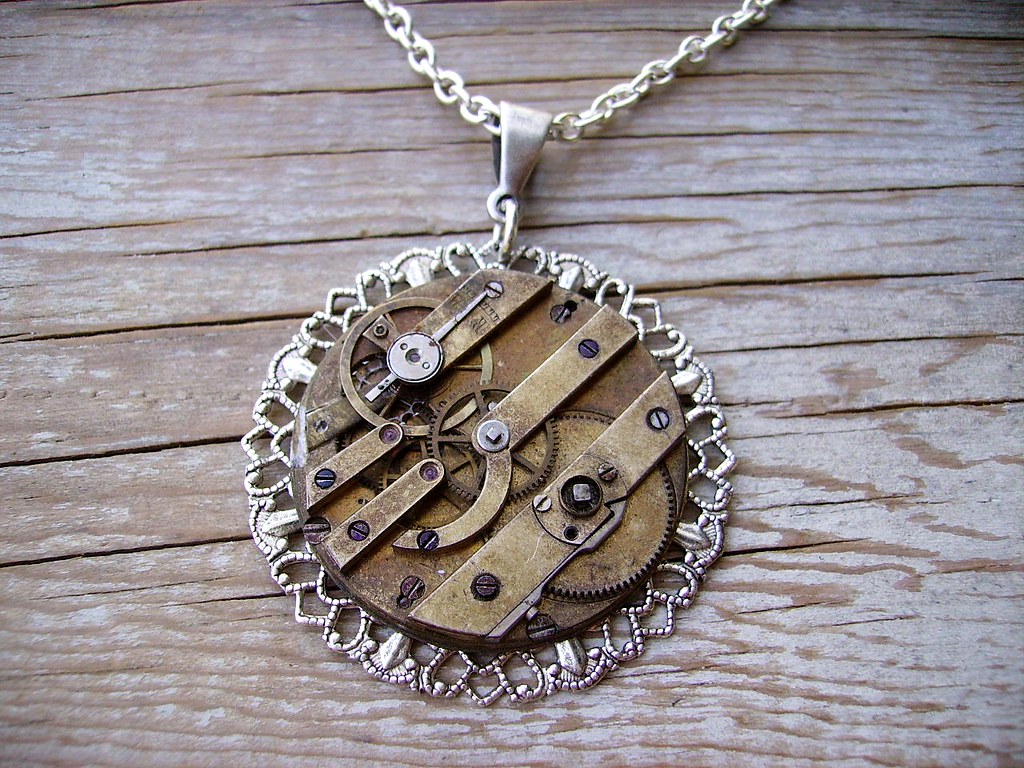The photograph depicts a close-up view of a distinctive, circular pendant necklace lying on a weathered wooden surface. The outer perimeter of the pendant features intricate, patterned metalwork in silver, forming a detailed, woven border. The centerpiece of the pendant is designed to resemble the intricate mechanisms of an old-fashioned watch, showcasing several interconnected gears and screws in shades of silver, brown, and copper. This mechanical design adds a vintage, steampunk vibe to the piece. The necklace is attached to a silver chain by a matching silver clasp, resembling the type commonly used in door security chains. The wooden surface beneath the necklace is light brown with black lines, appearing worn and slightly whitewashed, adding texture and depth to the composition. No other items are present in the image, allowing full focus on the detailed craftsmanship of the pendant.